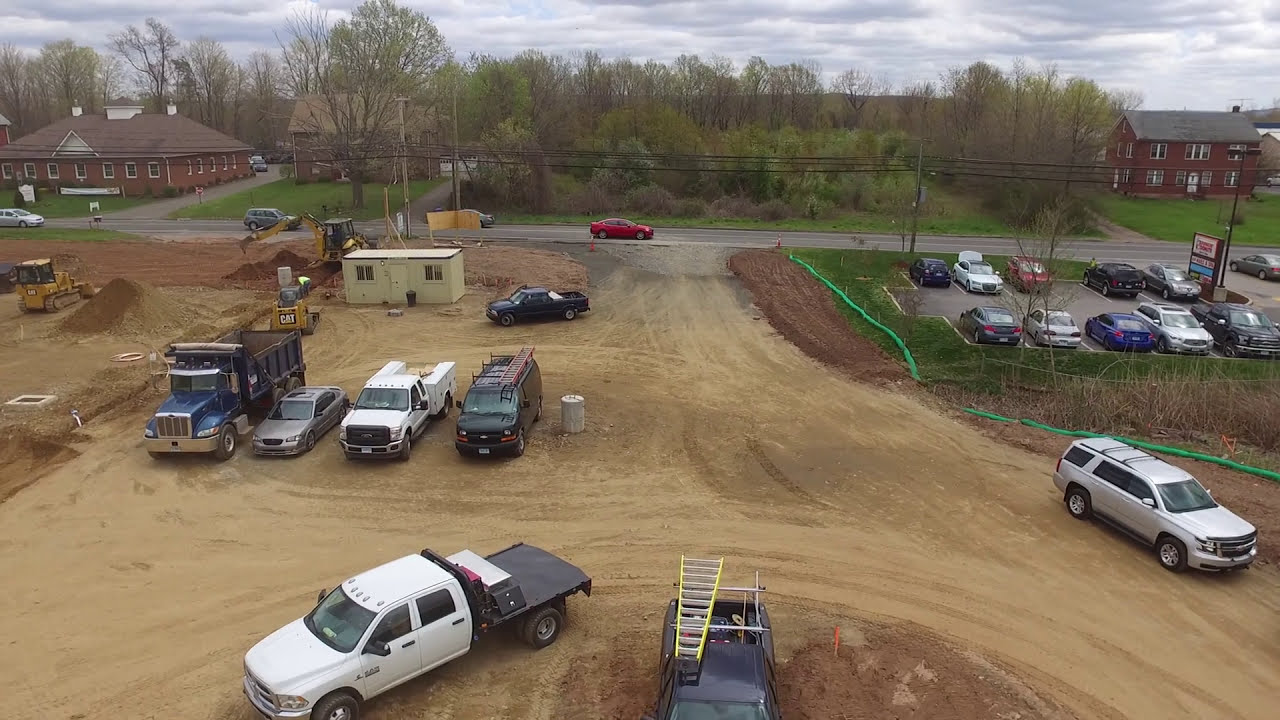The photograph captures an aerial view, possibly from a two or three-story building, overlooking a bustling construction site. Centered in the image is a dirt parking lot populated with an array of vehicles, prominently featuring two pickup trucks at the bottom center—one black with a yellow and gray ladder on top and another white flatbed with a toolbox. Adding to the scene’s industrial atmosphere, there's a semi-permanent trailer suggestive of a construction office.

To the left, several other vehicles are parked in a row, including a van, a white truck, a gray sedan, and a blue dump truck. Adjacent to these is a yellow tractor and various pieces of construction equipment, highlighting the active nature of the site, with bulldozers and dirt pushers maneuvering around a noticeable mound of dirt.

The dirt expanse seamlessly opens into a paved road running horizontally across the upper portion of the image, bordered by power lines. Beyond this road lies another parking lot, presumably for an existing business, with a visible Dunkin’ Donuts sign suggesting a commercial area. The backdrop features a mix of red brick buildings, possibly houses or businesses, intertwined with abundant greenery. The overcast, gray sky serves as a somber canopy over this vivid scene.